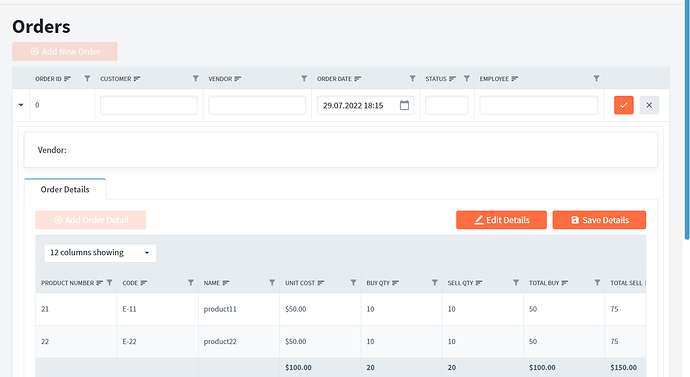Screenshot of an order page with detailed sections. The top half displays the customer’s name with an editable field, the vendor, the order date, the status, and the employee responsible. Two selectable options are visible: an orange check box and a gray X box. Below this, the order details include eight columns listing products, prices, and quantities. Users can edit and save these details. The page features three orange buttons for additional actions. The brand associated with the order is not specified.